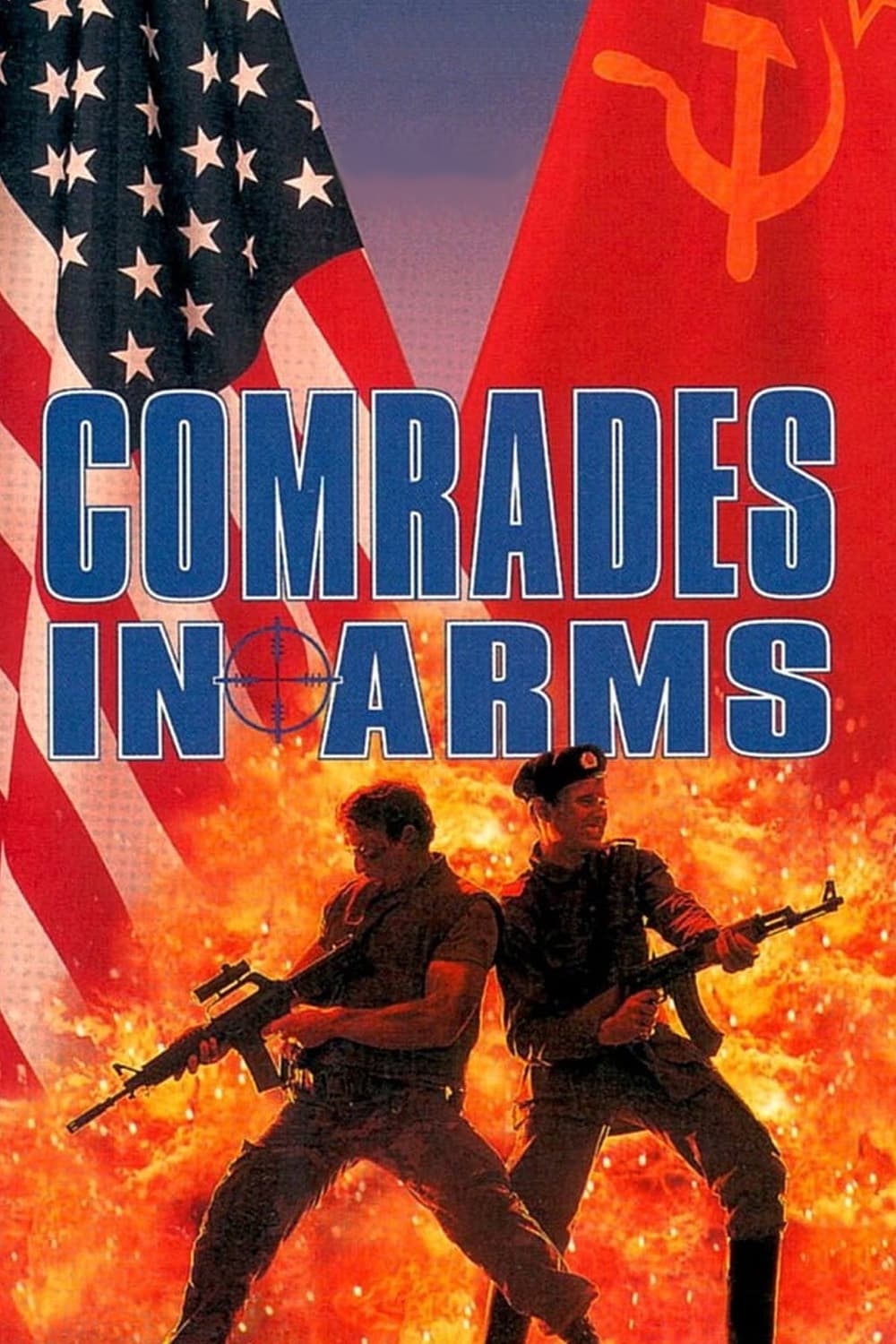The image is the cover of a book titled "Comrades in Arms," displayed prominently in blue text with a white border in the middle of the image. Between the words "in" and "arms," there's a scope sight symbol, also in blue. The cover is visually divided into two halves: the left side features a large American flag extending from the upper left corner towards the center, and the right side displays a large Soviet flag stretching from the upper right corner towards the center. Beneath the title are two white male soldiers, each holding assault rifles; the soldier on the left aims his rifle to the left, while the soldier on the right, who is wearing a beret, points his rifle to the right. Behind them is a dramatic backdrop of shooting flames, adding a red hue to the image and enhancing the intensity of the scene. The layout and dynamic elements suggest themes of conflict and camaraderie, fitting the book's title.